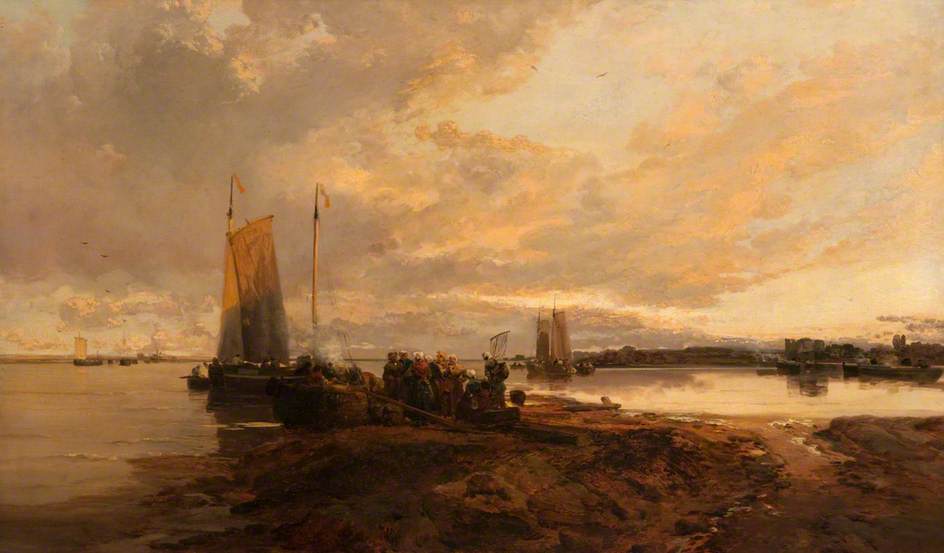The image showcases an intricately detailed oil on canvas painting depicting a historical seascape. This highly realistic painting captures a scene from what appears to be early evening, characterized by its use of muted tones and an overcast sky imbued with hues of orange and gray. The horizon is dominated by a vast expanse of water, likely a lake or ocean, dotted with several 17th-century sailboats. The focal point of the painting is a small sailboat positioned close to the shoreline, where a group of people, dressed in historical costumes, are either boarding or disembarking. The land along the water's edge is composed of brown, clay-like earth with debris rather than sandy beach, creating a sense of historical authenticity. Far in the distance, additional boats with small sails can be seen against the serene expanse of water. The overall atmosphere hints at the time of day being either early morning or late afternoon, suggested by the low daylight and the soft, natural colors reflecting a tranquil yet busy maritime scene.